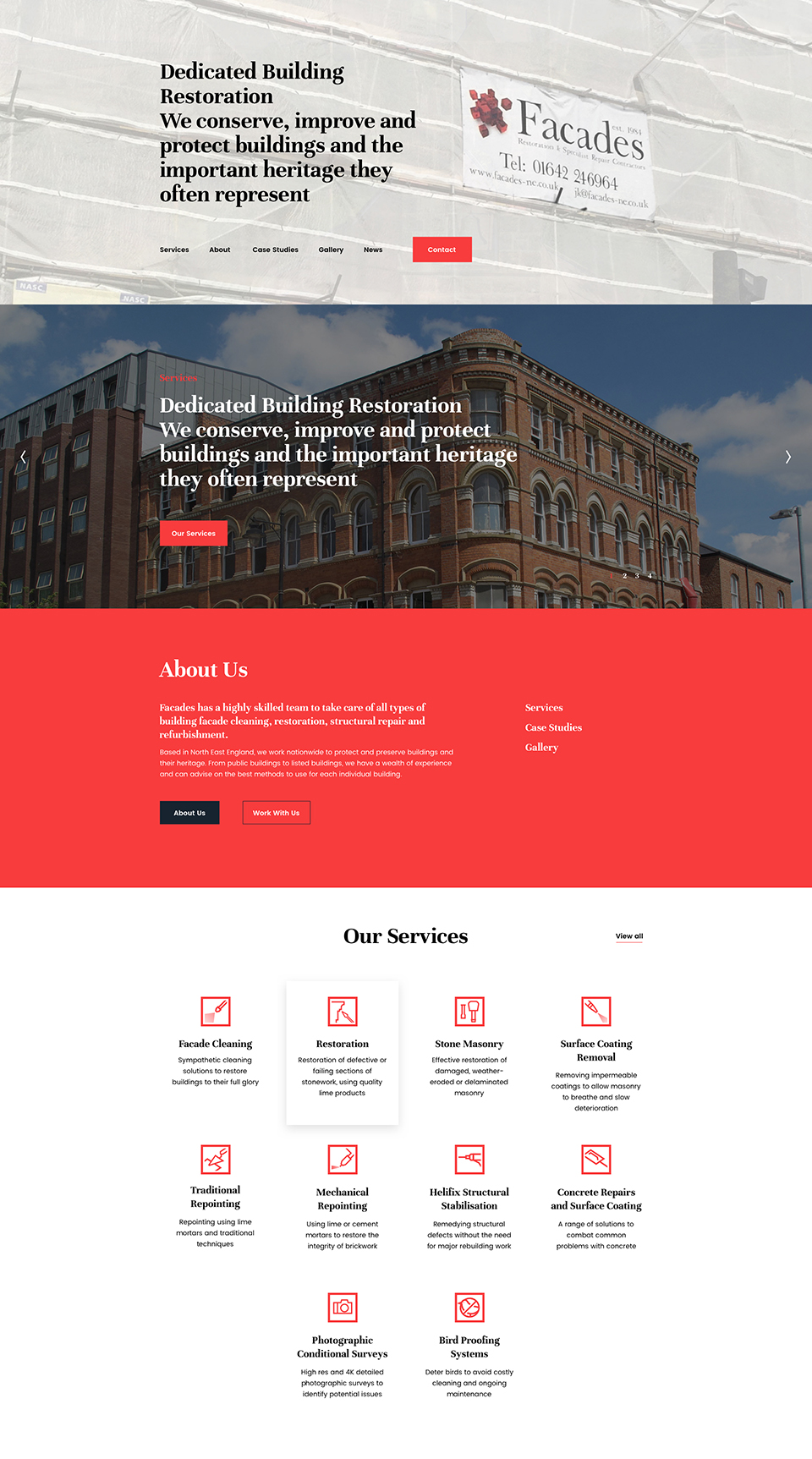In this close-up photograph of the FACADS website, the top section is prominently dominated by a banner or flag-like element that stretches across the width of the image, from left to right. This banner, which appears to be made of cloth and has a white background, nearly reaches the center of the visual frame. On the banner, there is a small tag featuring the text "FACADS" and a telephone number beneath it. To the right of this tag, the words "Dedicated Building Restoration: We conserve, improve, and protect buildings and the important heritage they often represent" are clearly displayed. Below this banner, a horizontal menu is visible. Further down, the image showcases a picture of a building accompanied by white text overlaid with a striking red button.